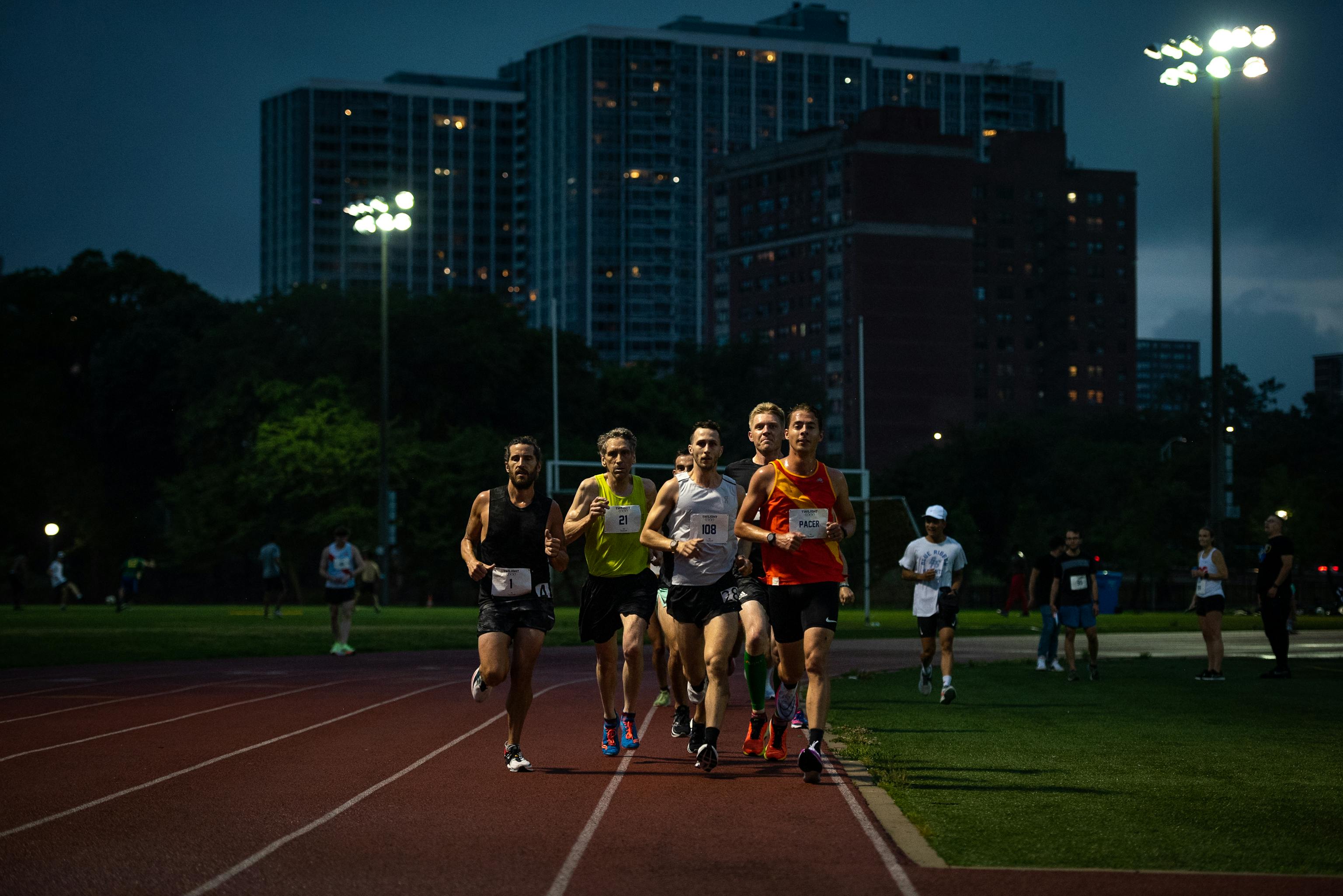This detailed nighttime photograph captures a group of runners on an outdoor track and field course. The image prominently features six runners in the foreground, with more partially visible behind them, suggesting a larger pack. They are racing on the inside lanes, indicating a distance event rather than a sprint, and are all clad in tank tops, running shorts, and gym shoes with short socks. Each runner has a number bib pinned to their chest or stomach area.

Illuminated by two towering light posts with multiple lights, the scene is bathed in bright artificial light, casting distinct shadows and revealing vivid details. The track itself is a rich brown with light gray stripes marking the lanes. The runners, emerging from a curve and heading straight toward the camera, are surrounded by spectators standing on the grassy infield and outer areas, attentively watching the race.

In the background, a large multi-story building looms, likely an apartment complex or an office tower, accompanied by a smaller building and a bank of shadowy green trees. Overhead, the sky is a deep blue, transitioning into night with patches of remaining daylight peeking through overcast clouds. The setting exudes the vibrant, focused energy of a night-time athletic event.